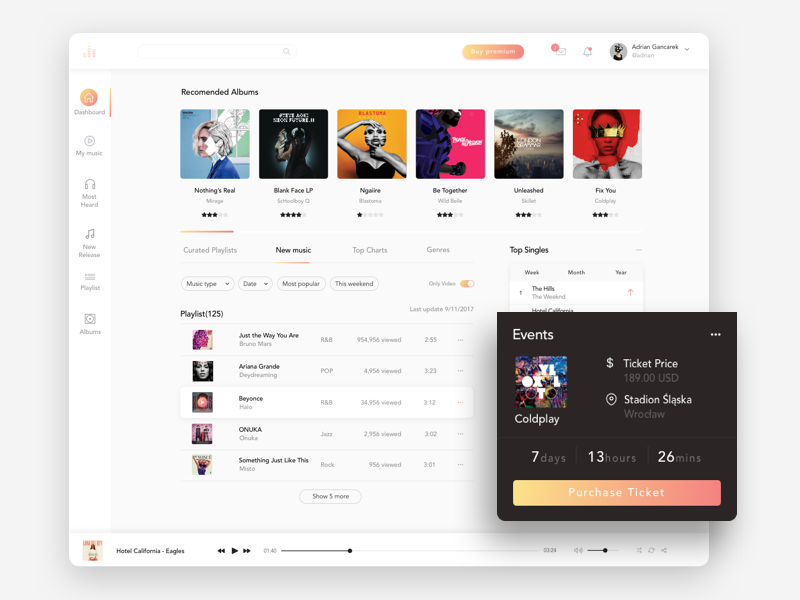The image depicts a dynamic user interface, possibly from a music streaming service or event app. In the bottom right corner, a black box prominently displays the word "Events," followed by "Coldplay," indicating an upcoming event for the renowned band. Below this, the ticket price is listed as $159 USD. The event is set to take place at Stadion Śląski, with a countdown timer indicating 7 days, 13 hours, and 26 minutes remaining until the event, along with an option to purchase a ticket highlighted in a vibrant yellow, orange, and pink rectangle.

At the top of the interface, there's a section labeled "Recommended Albums," featuring small album illustrations with titles beneath them. Identifiable albums include "Fix You" by Coldplay, "Nothing's Real," "Blank Face LP," "Be Together," and "Unleashed." Despite their reduced size, the illustrations add a visual appeal to the section.

In the upper left corner, an orange-colored house icon marks the start of a navigation menu, listing options such as "Dashboard," "My Music," "Most Heard," "New Releases," "Playlists," and "Albums." Finally, at the very bottom of the screen, there's a mention of "Hotel California" by The Eagles, along with an option to play the track. The detailed layout and vibrant colors of the interface make it user-friendly and visually engaging.